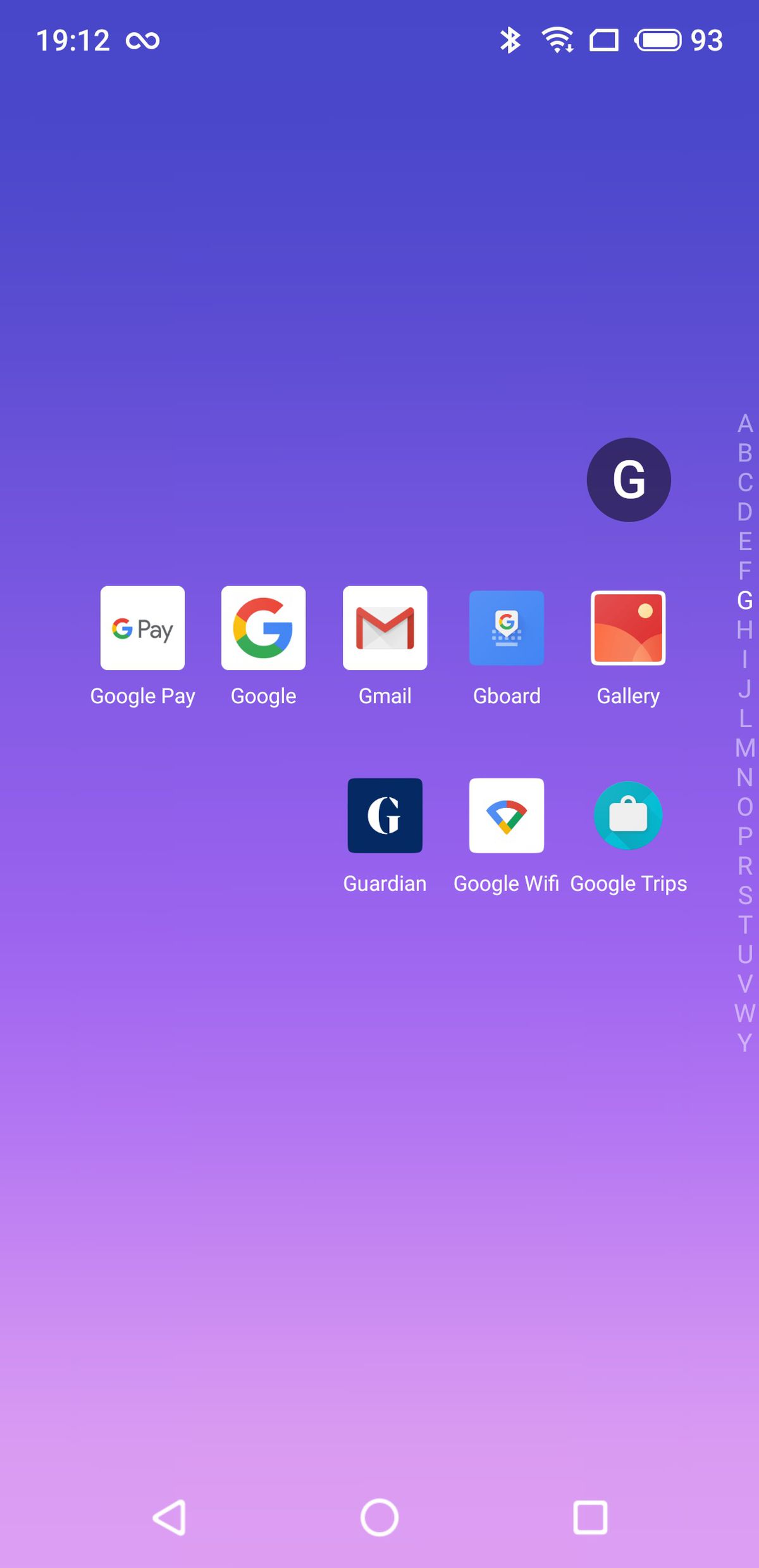The image features a gradient background that transitions from a purplish tint at the top to a pinkish hue at the bottom, with a bluish tint in between. On the left side, the display shows the time "19:12," along with an indication of no cellular bars, and a battery life of 93%. Running vertically down the right side of the image is the alphabet, from "A" to "Y." 

Adjacent to the right side alphabet is a column of icons and text. At the top of this column is the letter "G" enclosed within an oval shape, followed by a row of five squares. Each square contains a label and a logo: 
1. "Google Pay" with its respective logo.
2. "Google" with its logo.
3. "Gmail" with its logo.
4. "Gboard" with its logo.
5. "Gallery" with its logo.

Below these squares is a row of three additional icons, labeled:
1. "Guardian" with its corresponding logo.
2. "Google Wi-Fi" with its logo.
3. "Google Trips" with its logo.

At the bottom of the image, there are four control buttons: a "Play" button, a "Pause" button, a "Record" button, and a "Stop" button.